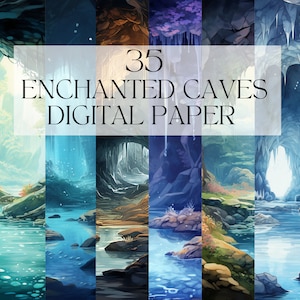The image serves as an advertisement, likely for the front of a box or a digital planner cover, titled "35 Enchanted Caves Digital Papers." It prominently features six vertical panels, each showcasing a distinct fantasy cave environment. The first panel depicts a scene with green water, a blue sky, and some ground. The next panel illustrates a dark river flanked by rocks and a forest. The third panel shows an opening in a cave that leads to blue water and a forest beyond. The fourth panel presents blue water accompanied by purple plants in a dark cave. Following that, the fifth panel highlights a landscape with brown rocks, green grass, and clouds in the background. The final panel displays an underground cave with stalagmites hanging from the ceiling and an opening leading to water. All six panels share a similar magical and otherworldly aesthetic, capturing different elements of enchanting cave environments. The only text on the image is the title, "35 Enchanted Caves Digital Papers," which appears as a white watermark, emphasizing its purpose as a product advertisement.